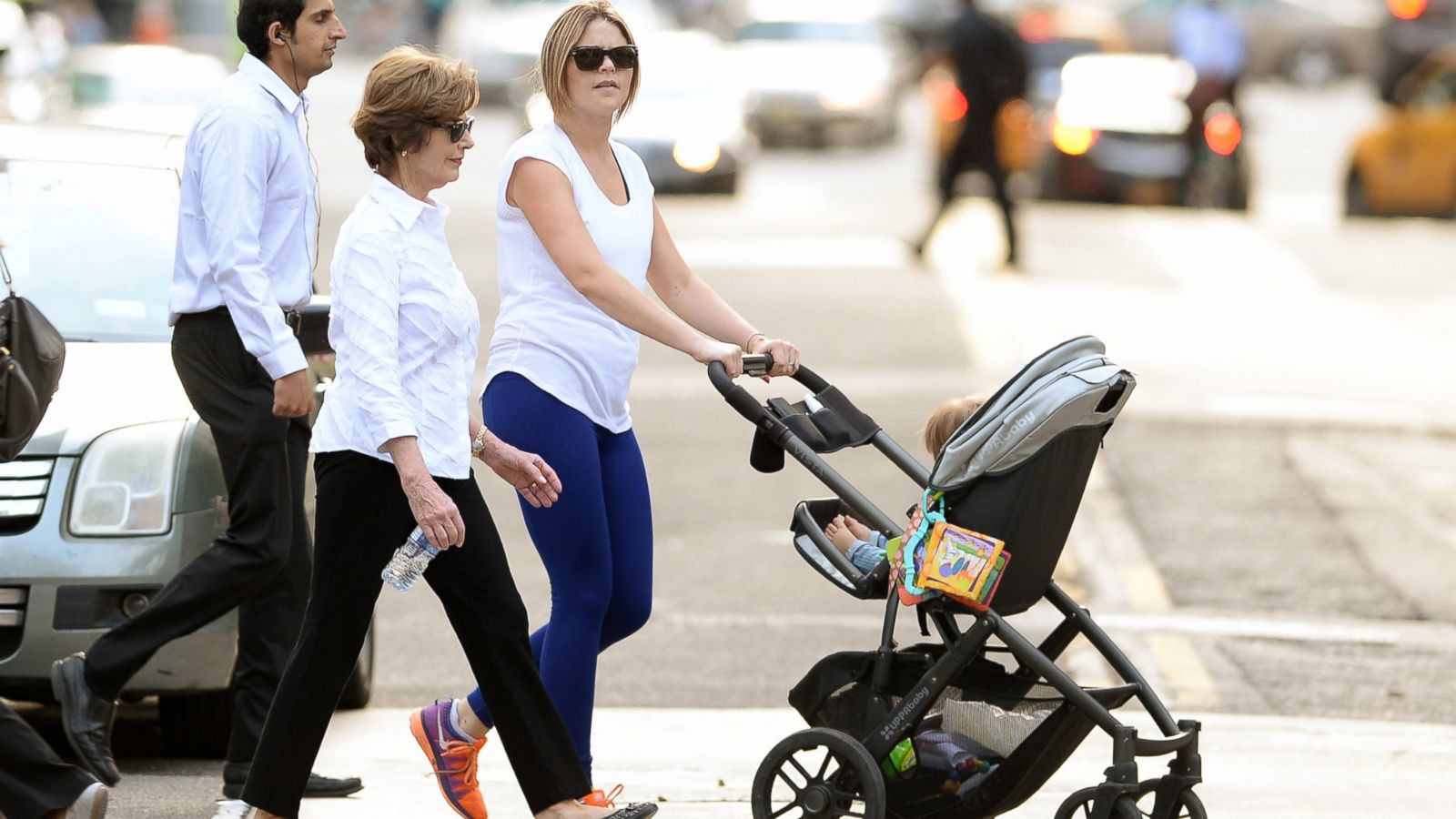In this lively urban scene, three individuals are walking across a busy city street filled with parked cars, some of which are blurred into the background. The woman in the center of the group is pushing a stroller that holds a small child, whose tiny feet in a onesie are visible, while the stroller's basket beneath is filled with various baby essentials like diapers, a bag of baby wipes, and some children's playbooks attached to the side. She is dressed in a white tank top, blue leggings, and sneakers, and wears sunglasses, giving a somewhat indifferent look towards the camera. 

To her right is an older woman, also in sunglasses, focused straight ahead. She is dressed in a white buttoned-up long-sleeve shirt, black pants, and holds a water bottle in one hand. She also has a gold watch and a wedding ring on her left wrist. 

Behind the woman with the stroller walks a man in business attire: a white buttoned-up shirt tucked into black dress pants, complemented by dress shoes and a belt. He has a Bluetooth headset in his ears and his eyes are closed as he walks. Together, these three individuals, seemingly strangers, navigate the city crosswalk towards their separate destinations.